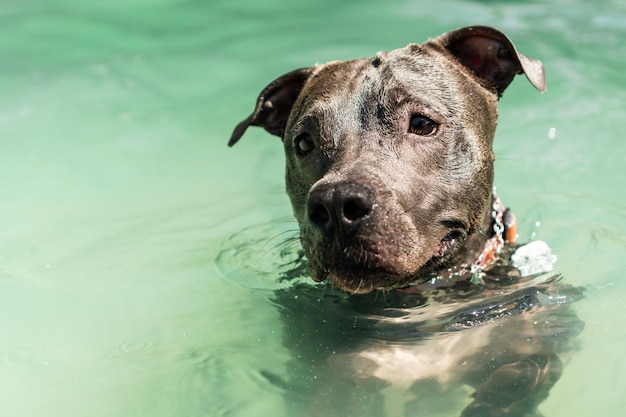The photograph captures a dog, identified as a pit bull-lab mix, swimming forward in water that has a greenish-blue hue, making the tan-colored bottom slightly visible through its clear surface. The dog, characterized by a brown face and back with a white chest, is adorned with a metal chain collar and an adjustable orange canvas collar. With its floppy ears and a big black nose, the dog’s dark eyes are not looking at the camera but rather off-screen towards the top left, giving an impression of sadness or unease. The head of the dog creates ripples in the water, and you can see part of its body and legs submerged. The scene is focused solely on the dog, leaving the nature of the water—whether a natural body or a pool—ambiguous.